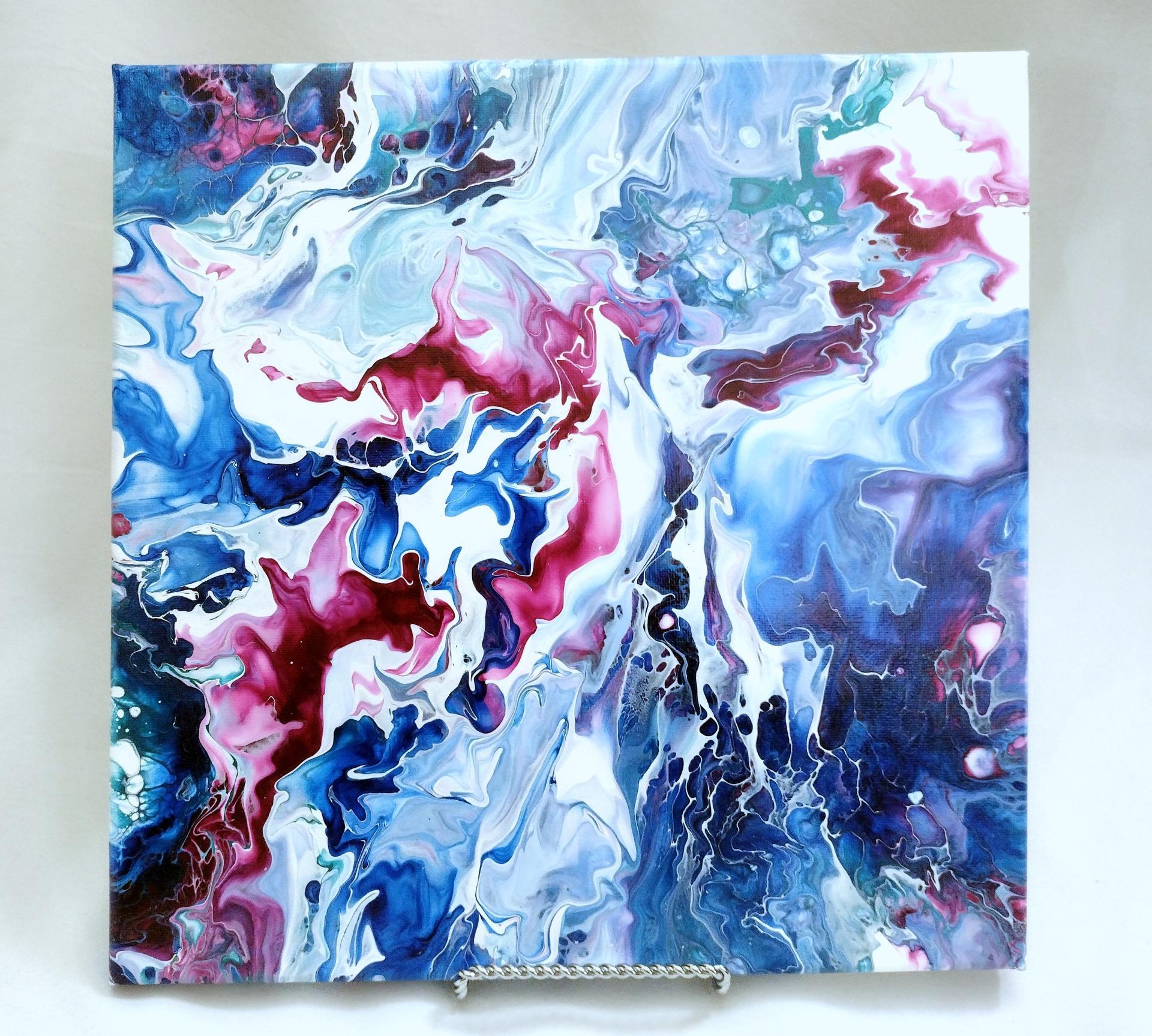This photograph captures an abstract painting, possibly on canvas, hanging prominently on a wall, which transitions from gray on the left and top to white towards the middle and bottom right due to shadow play. The painting itself, square in shape and colorful, is supported by a slender, silver horizontal rod with a delicate spiral metal design, positioned at the bottom. The artwork is characterized by its dynamic swirls and blobs of vibrant colors, ranging from dark and light blues, maroons, dark reds, pinks, purples, greens, to whites and grays. The lower section of the painting is dominated by shades of dark blue, maroon, dark red, and pink, which swirl upwards towards the predominantly purple, white, and light blue middle section. Lighter hues like pale blues, greens, grays, and pinks populate the upper part, with a mix of darker blues and hints of purple in the upper left corner. The fuchsia-colored swirls extend from the lower left to the middle, giving the painting a somewhat floral but distinctly abstract appearance. The image seems to occupy most of the artwork, with a minimal off-white border visible around it, suggesting it might be displayed in an art museum.